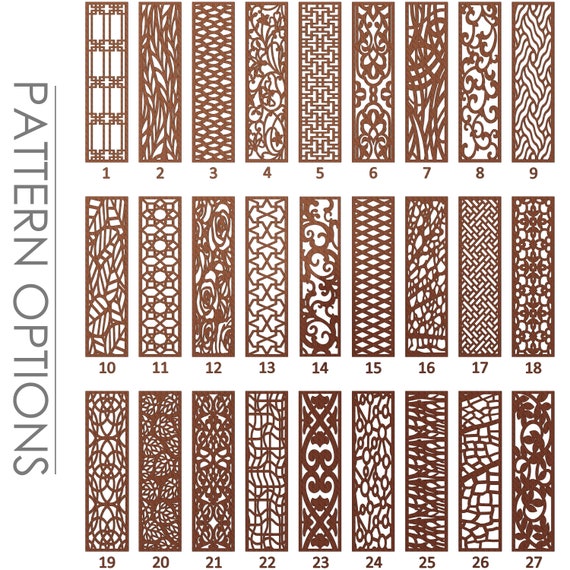The image is oriented in portrait vertical, displaying the phrase "PATTERN OPTIONS" in gray capital letters, rotated 90 degrees along the left edge. It features three rows of rectangular patterns, each row containing nine designs, numbered consecutively from 1 to 27. The patterns are displayed as brown designs on a white background. Notably, the second pattern resembles a cluster of leaves, the 15th pattern has a crisscross fishnet design, and the 22nd pattern features a grid of vertical and horizontal lines forming rounded squares. Each pattern is distinct yet uniform in size, offering a variety of aesthetic options within the same dimensions.